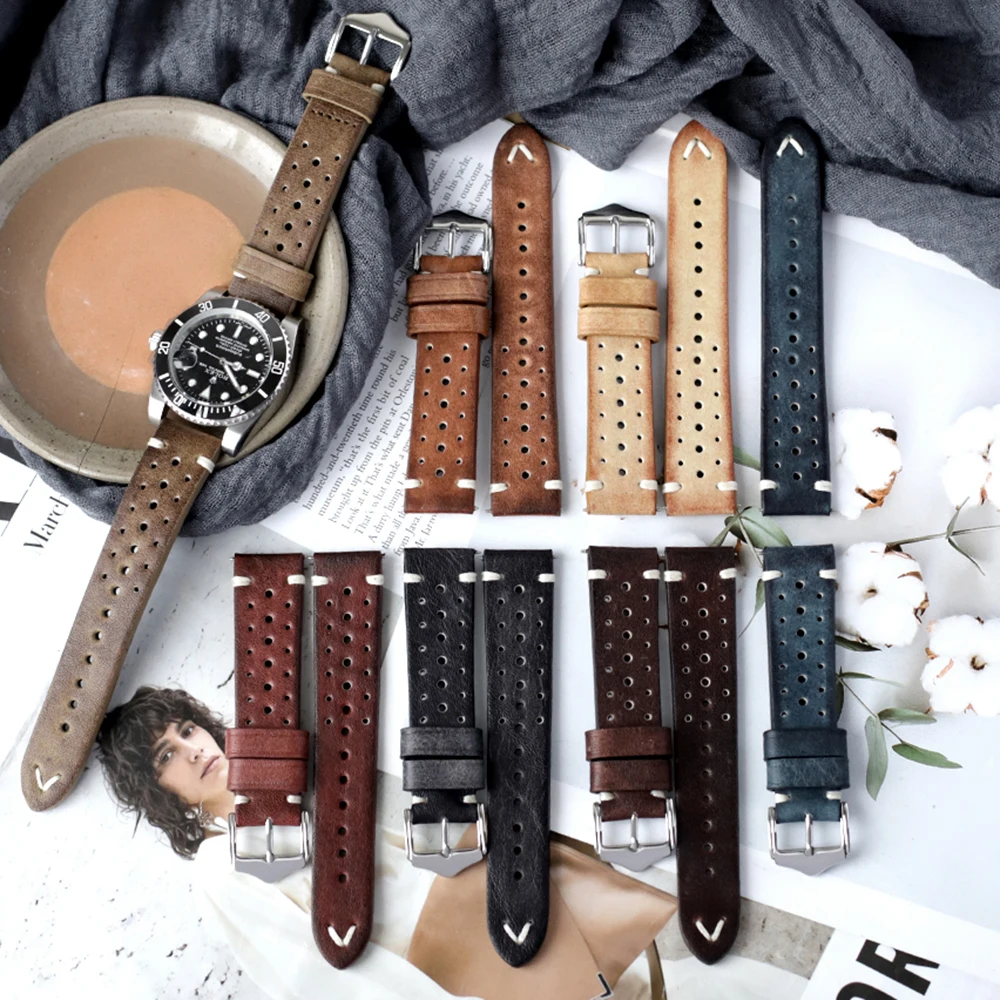In the upper portion of the image, there is a soft cloth that resembles a sheet or towel. Positioned on the upper left side is a round disc, which transitions in color from gray on the outer edge to brown and then to a light brown hue towards the center. Resting atop this disc is a watch with a silver face and black center. The watch features brown leather bands punctuated with holes. Surrounding the watch are several other leather bands in various colors: dark brown, beige, and gray. At the bottom of the image, additional leather bands are visible in burgundy, charcoal gray, and an extremely dark brown shade, along with another segment of gray. Overlapping a partially visible magazine page in the lower left corner is an image of a woman with brown hair, carrying a beige bag. On the right side of the magazine page, near the leather bands, there are unreadable words; the only discernible text reads "at."